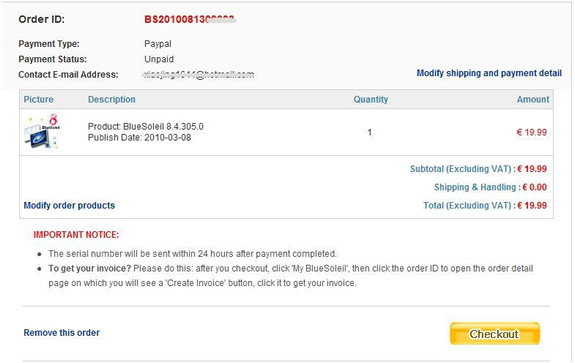"An image of an order form detailing a purchase transaction is shown. The form includes the following sections:

1. **Payment Type:** Listed as 'PayPal'
2. **Payment Status:** Marked as 'Unpaid'
3. **Order ID Number:** Displayed prominently
4. **Product Image:** A visual representation of the ordered item
5. **Price Information:**
   - Listed Price: €19.99
   - Subtotal: €19.99
   - Shipping and Handling: €0
   - Total: €19.99

**Additional Details:**
- The ordered item is categorized under 'Modified Water Products.'
- An important notice indicates that the serial number will be sent to the buyer, with instructions to ensure the checking process is completed to receive the invoice.
- A yellow 'Checkout' bar is prominently displayed at the bottom.
- The total amount is written in red, while all other text is in blue."